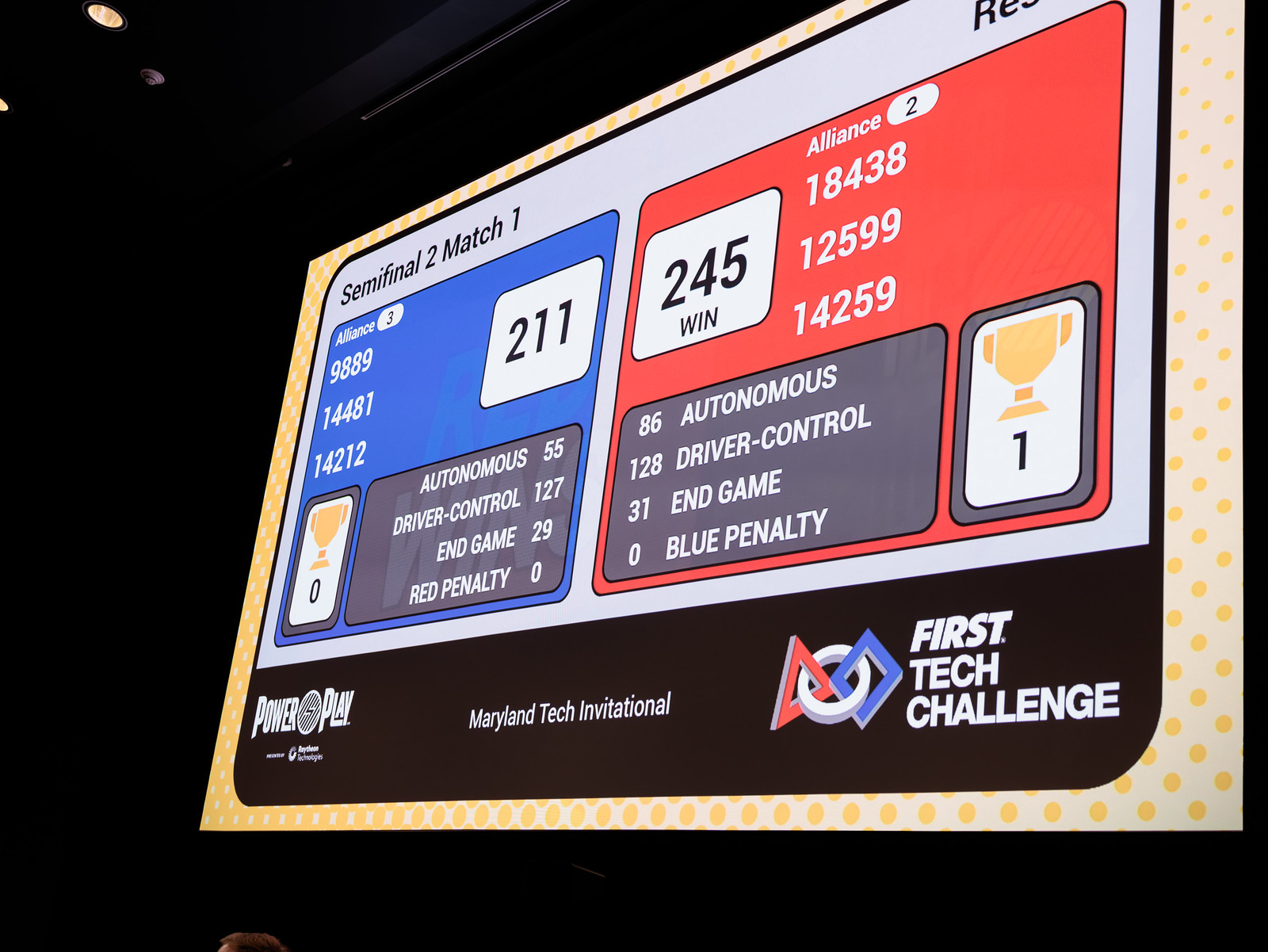The image depicts a brightly lit scoreboard set against a black background, displaying the results of a competition titled "Maryland Tech Invitational" with a logo indicating it's part of the "First Tech Challenge" and themed "Power Play." The scoreboard is divided into two sections: on the left side, which has a blue background, it shows the results for the blue team. It reads "Semi-finals 2, Match 1," and shows the score breakdown into categories: "Autonomous 55," "Driver Control 127," "End Game 29," and "Red Penalty 0." The total score for the blue team is "211," indicating a loss. The blue section also lists "Alliance 3" with team numbers "9889, 14481, 14212."

On the right side, with a red background, it displays the red team's score as "245 Win." The breakdown includes "Autonomous 86," "Driver Control 128," "End Game 31," and "Blue Penalty 0." This section lists "Alliance 2," featuring teams "18438, 12599, 14259." Underneath the scores, a small trophy icon indicates the red team has one win. The entire screen is framed and features yellow dots around the perimeter, creating a highlighted effect, while the rest of the image remains in darkness.